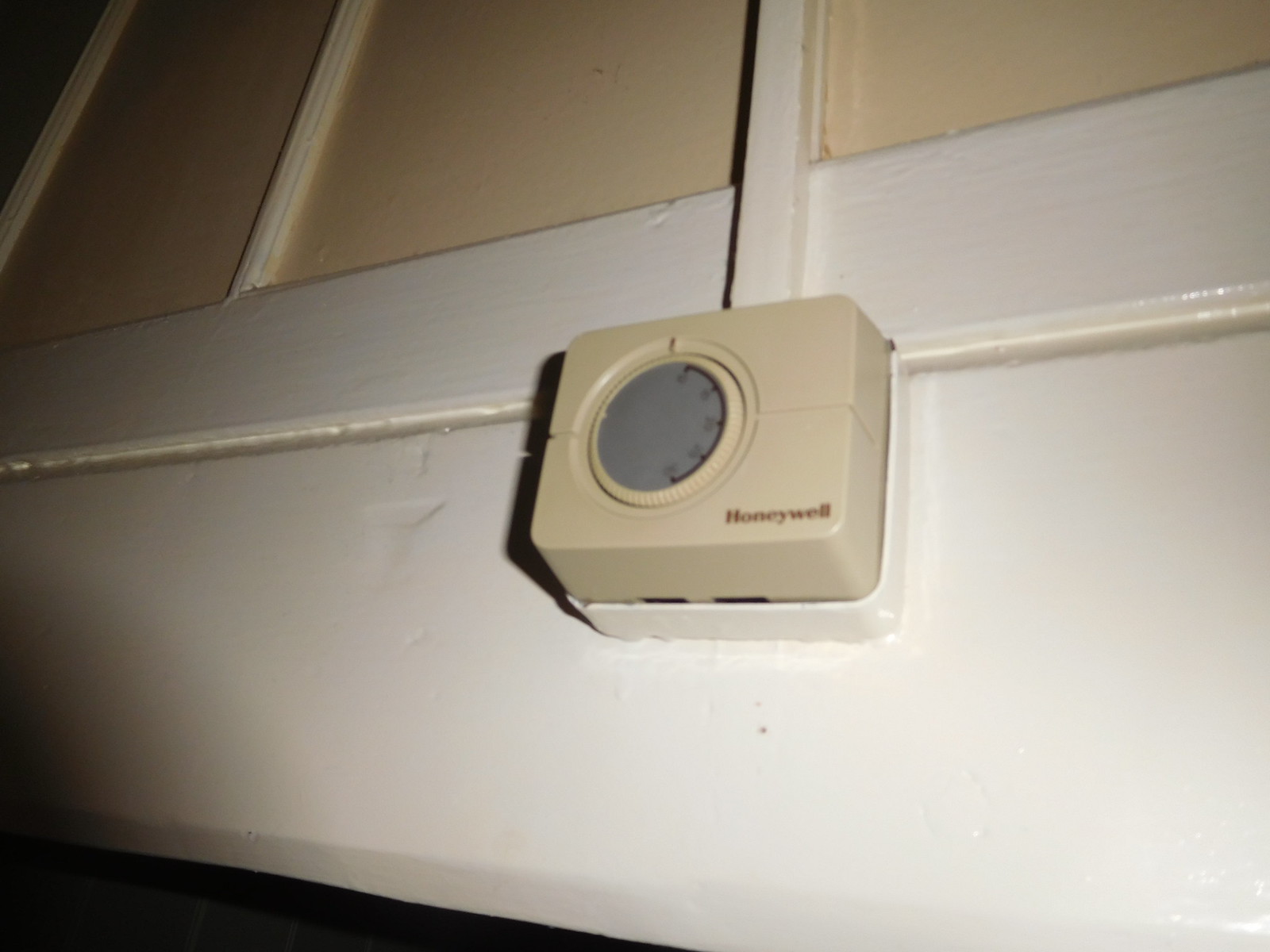This image captures the lower section of a house's interior wall, featuring a detailed view of the baseboard and adjacent wall. The white baseboard runs horizontally along the bottom, with dark shadows visible in the bottom left corner of the frame, suggesting low ambient light conditions. Above the baseboard, the wall is painted a beige-tan color, adorned with vertical white molding stripes spaced approximately 6 to 8 inches apart, creating a decorative pattern. 

Central to the composition is a long vertical molding strip that seamlessly transitions into a beige-colored box, which is mounted on the wall. The box, identified as a Honeywell device, features a front dial with numbered settings and sits atop a small white base. There is a horizontal etching just above the baseboard, which spans the entire width of the image, giving the appearance of an intentional design element carved into the wood. The upper left corner of the photo is slightly darker than the rest of the illuminated wall, likely due to the directional lighting provided by a camera flash.